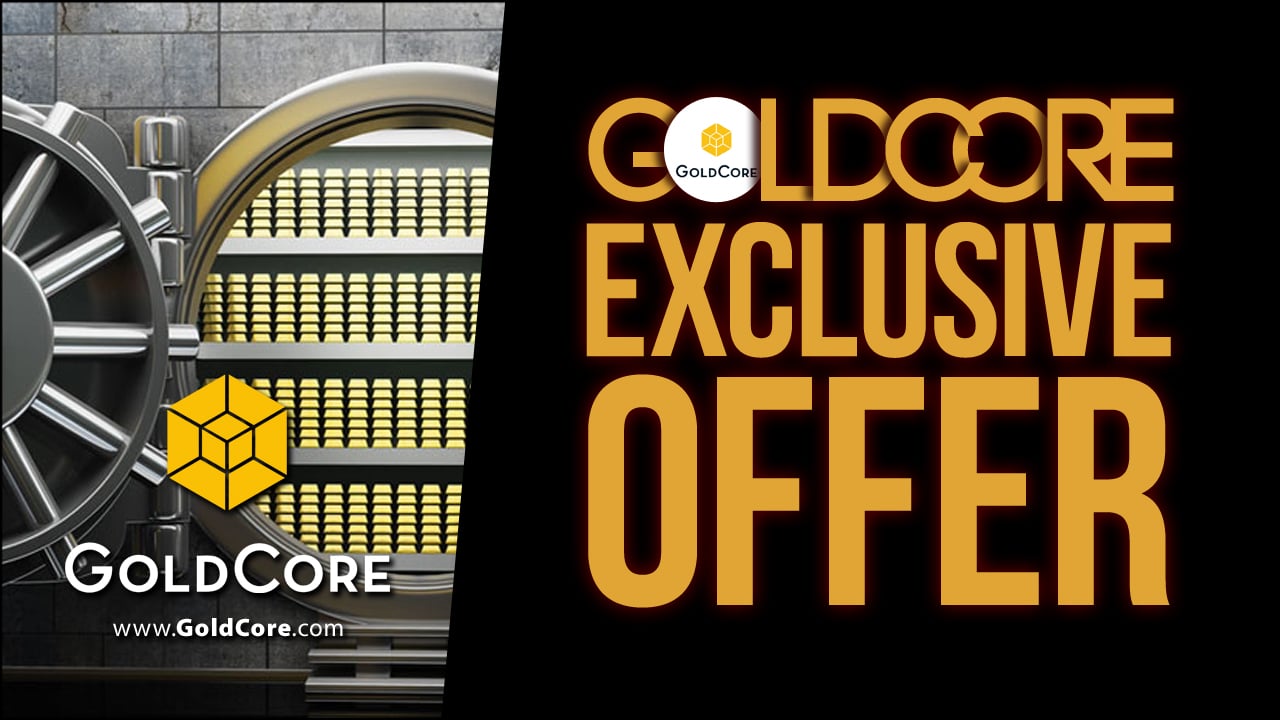This advertisement showcases GoldCore's exclusive offer. Dominating the image are gigantic gold letters spelling "GoldCore Exclusive Offer" on a black background, with the distinctive GoldCore logo—an interlocking gold cube—integrated into the letter "O" of GoldCore. This bold text covers two-thirds of the advertisement. On the left side of the ad, a compelling depiction of a vault filled with meticulously stacked gold bars captures immediate attention. The GoldCore logo appears at the center of this vault image, accompanied by the website address, www.goldcore.com, displayed in white font at the bottom.